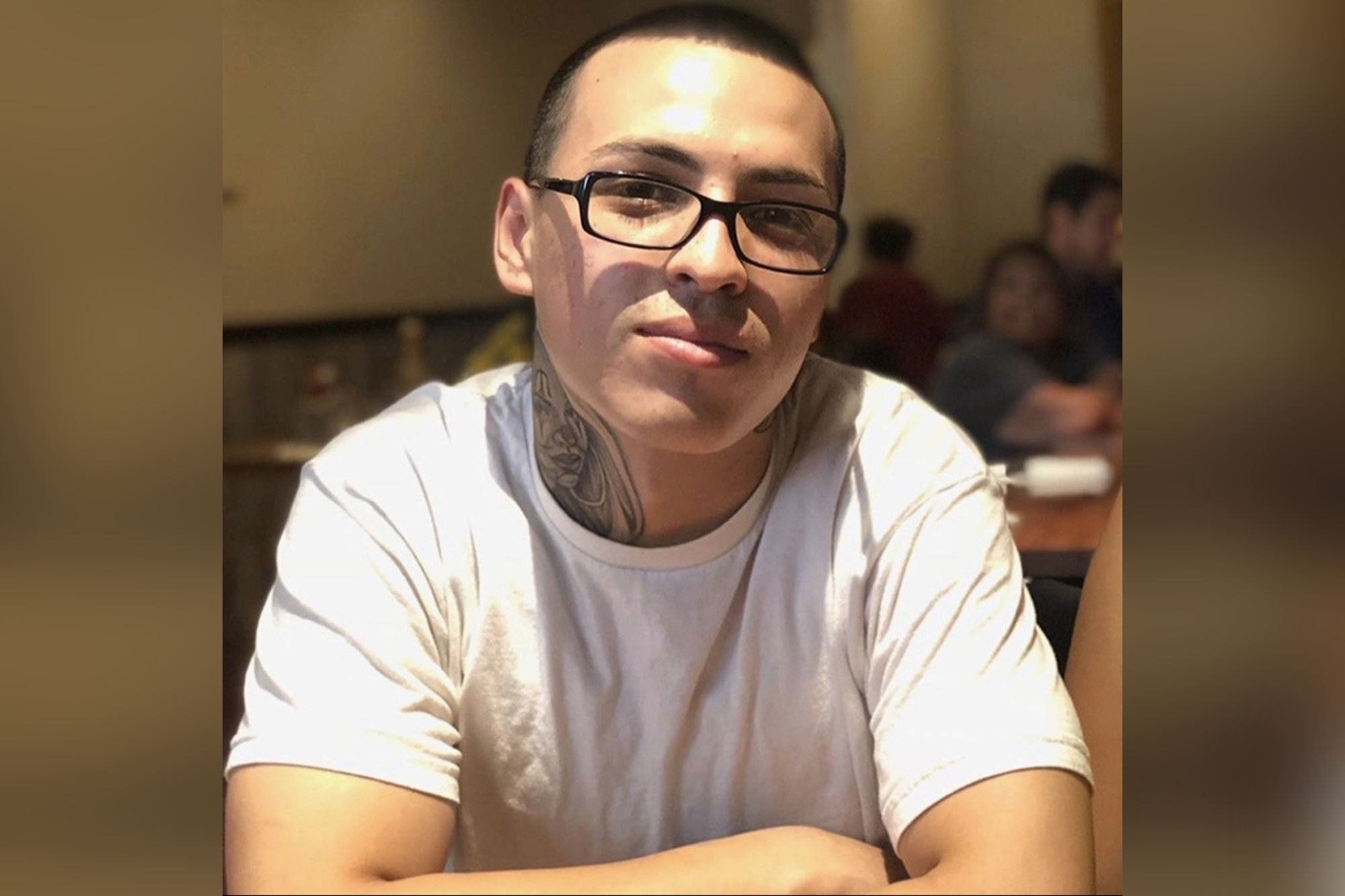The image features a young Hispanic man, likely in his mid-20s, seated at a table with his arms folded across his chest. He is wearing a white short-sleeved t-shirt and has dark black-rimmed glasses. His hair is very short, nearly buzz-cut, and he sports a tattoo on the right side of his neck that resembles a girl's face. He appears to be slightly smirking, giving the impression of discomfort with having his photo taken. The background shows a few indistinct figures sitting in the distance, their features blurred out. The setting is a room with white-colored walls, described variously as dark and colorless, contributing to a somewhat stark and unwelcoming atmosphere. The photograph is horizontally oriented and rectangular in shape.